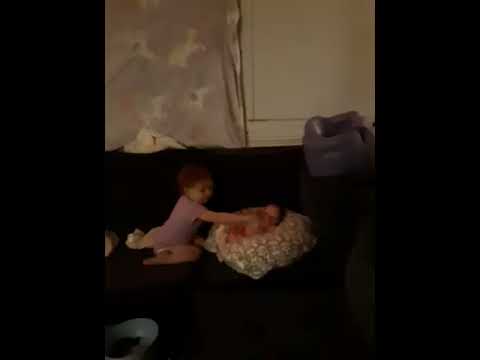In the image, a toddler with red hair, dressed in a light pink short-sleeved t-shirt, sits on the ground on the left side, smiling and interacting with an infant next to them. The infant, lying in an ornamental basket adorned with a lace cloth and flowers, has dark hair and is nestled comfortably. The setting appears to aim for a photo shoot feel, with the blanket around the baby being adjusted by the toddler and the dark carpeted floor adding contrast. Behind the children, a gray fabric featuring white patterns hangs on the wall, next to a white wall. In the upper right corner, there is a gray baby or toddler chair visible, adding to the cozy indoor environment. This harmonious scene captures a tender moment shared between the two young children.